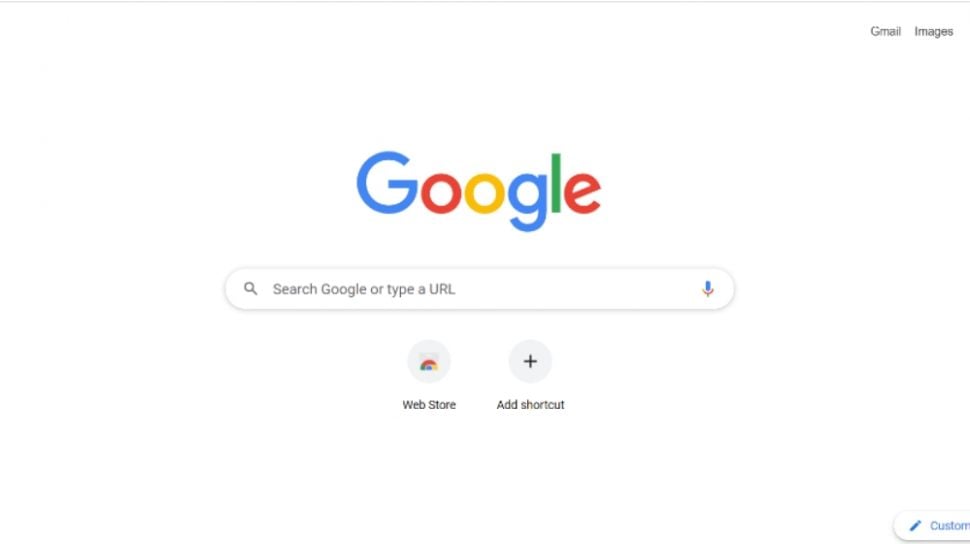The image depicts a classic Google search homepage against a large white background. At the top of the page, there is a light gray line featuring the options "Gmail" and "Images" in gray text. In the center of the page, the iconic Google logo is prominently displayed, featuring a blue 'G', red 'O', yellow 'O', another blue 'G', a green 'L', and a red 'E'. Below the logo, there is a gray-bordered search box with a white interior prompting the user with the text "Search Google or type a URL". On the right side of the search box, there is a microphone icon colored in blue and red, indicative of Google’s voice search functionality.

On the homepage, there are two gray circles beneath the search box. The first circle has an icon composed of a red, yellow, and blue half-circle and is labeled "Web Store". The second circle features a plus sign and is marked "Add Shortcut". Towards the bottom right corner, there's an additional small gray box with a blue pencil icon labeled "Customize".

The overall layout allows users to search Google or enter a URL, access the web store, add shortcuts, or customize their search page, providing a streamlined and interactive user experience.